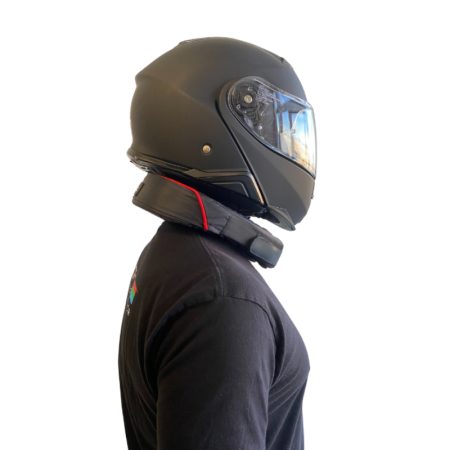This image features a side profile of an individual whose gender is ambiguous, wearing a sturdy, dark black motorcycle helmet with a clear plastic visor covering their eyes. The helmet envelops the entire head, including the chin and mouth, and is designed with a durable look suitable for riding motorcycles. Around the person’s neck, there is a black padded neck cushion adorned with a distinctive red line running along its back. The individual is clothed in a dark gray or black long-sleeved shirt, and a faint glimpse of a logo in red, green, and blue can be seen on the back of the shirt. The background of the image is a plain white, emphasizing the prominence of the person and their protective gear.